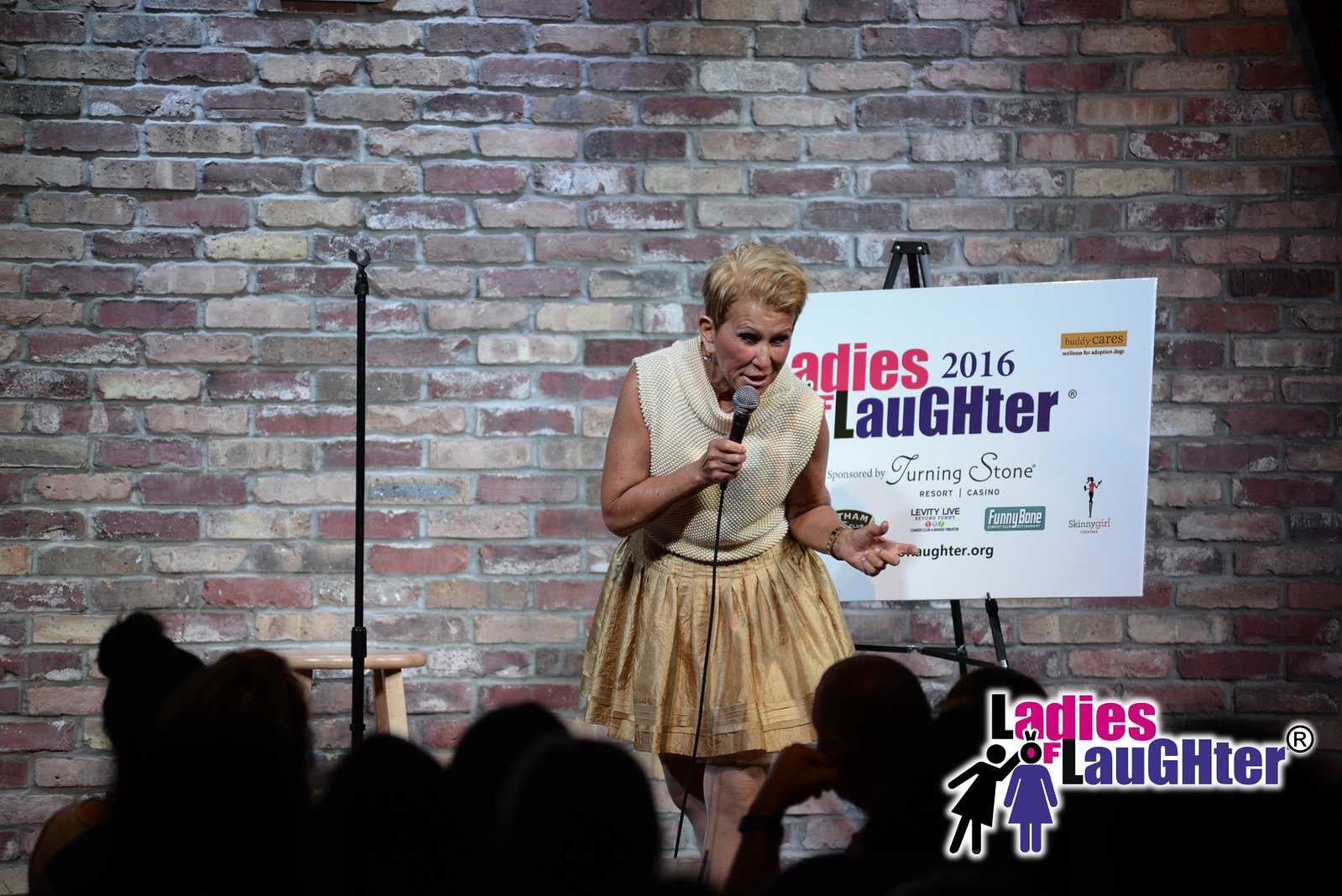The photograph captures a seasoned woman, likely in her fifties, leaning forward and speaking animatedly into a black microphone with a rounded top. She stands center stage in front of a textured, multicolored old brick wall, which ranges in shades from red to gray to beige, with visible gray mortar. Wearing a sleeveless white sweater top with a turtleneck and a knee-length short yellow skirt, she commands the small comedy club stage. Her blonde bleached hair is cropped short. To her left, a light brown wooden barstool stands next to a black microphone stand. Behind her, partially obscured, an easel holds a sign reading "Ladies of Laughter 2016, sponsored by Turning Stone Resort Casino." In the foreground, the silhouettes of the audience are faintly visible, while the bottom right corner of the image features a superimposed logo that reiterates "Ladies of Laughter." This detailed background and the speaker's commanding presence suggest the lively atmosphere of a comedy event.